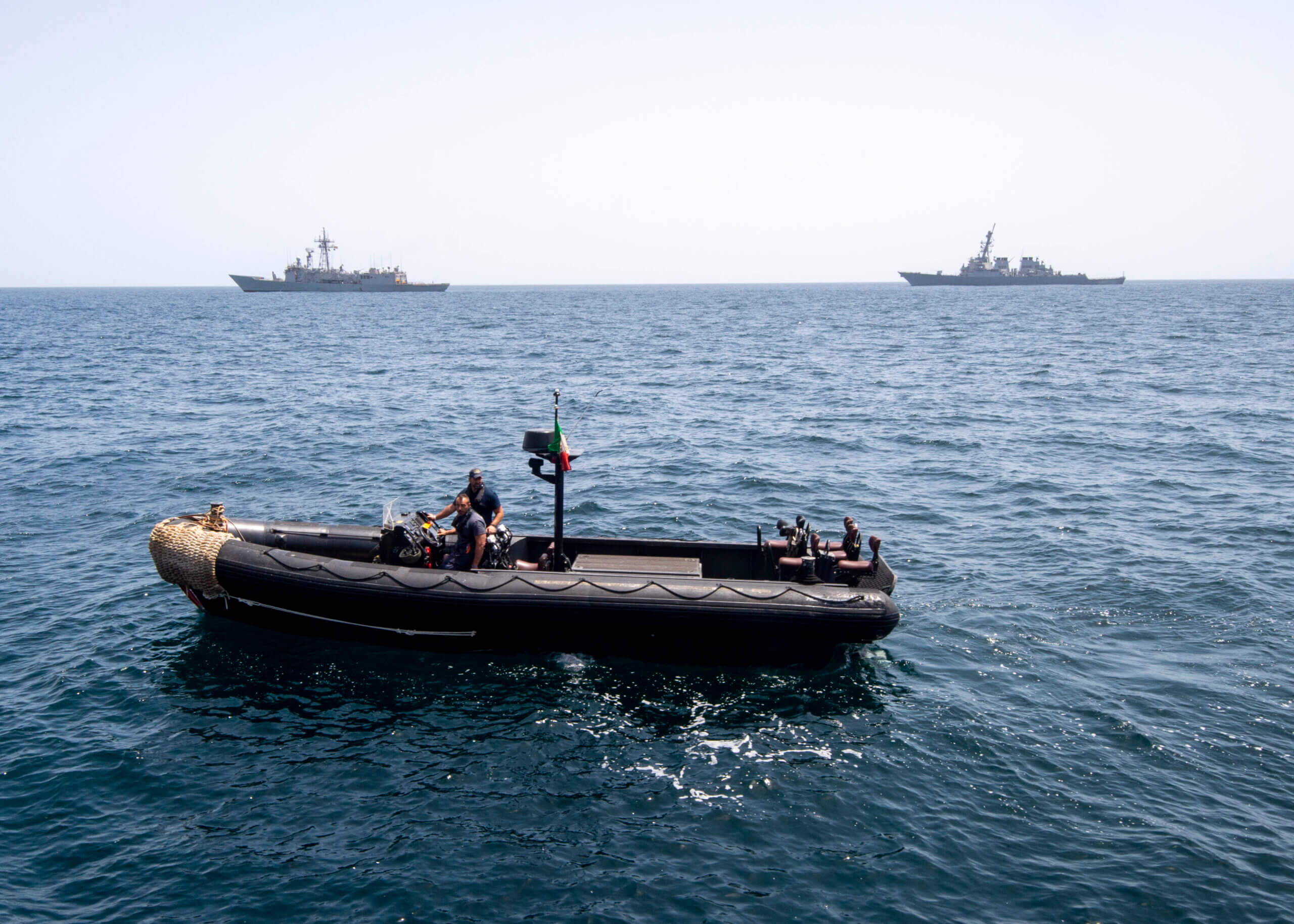In this photograph, we see a small boat navigating the calm, bright blue ocean. The focal point of the image is the two men, possibly soldiers, aboard this small vessel, which seems to be on an exploratory mission. A third person can be observed sitting in the back of the boat. The boat looks business-like with no visible weapons, possibly equipped with radar equipment. The backdrop of the scene includes two larger ships, likely battleships or cargo ships, situated one on the left and one on the right side of the photo. The day is cloudy with grey skies, suggesting the possibility of rain. Despite the overcast weather, the water remains serene, contrasting with the sky. The smaller boat might be part of a larger battalion associated with the bigger vessels, assisting in covering more ground rapidly. This detailed scene is clearly a real photograph, capturing a genuine moment on the ocean.